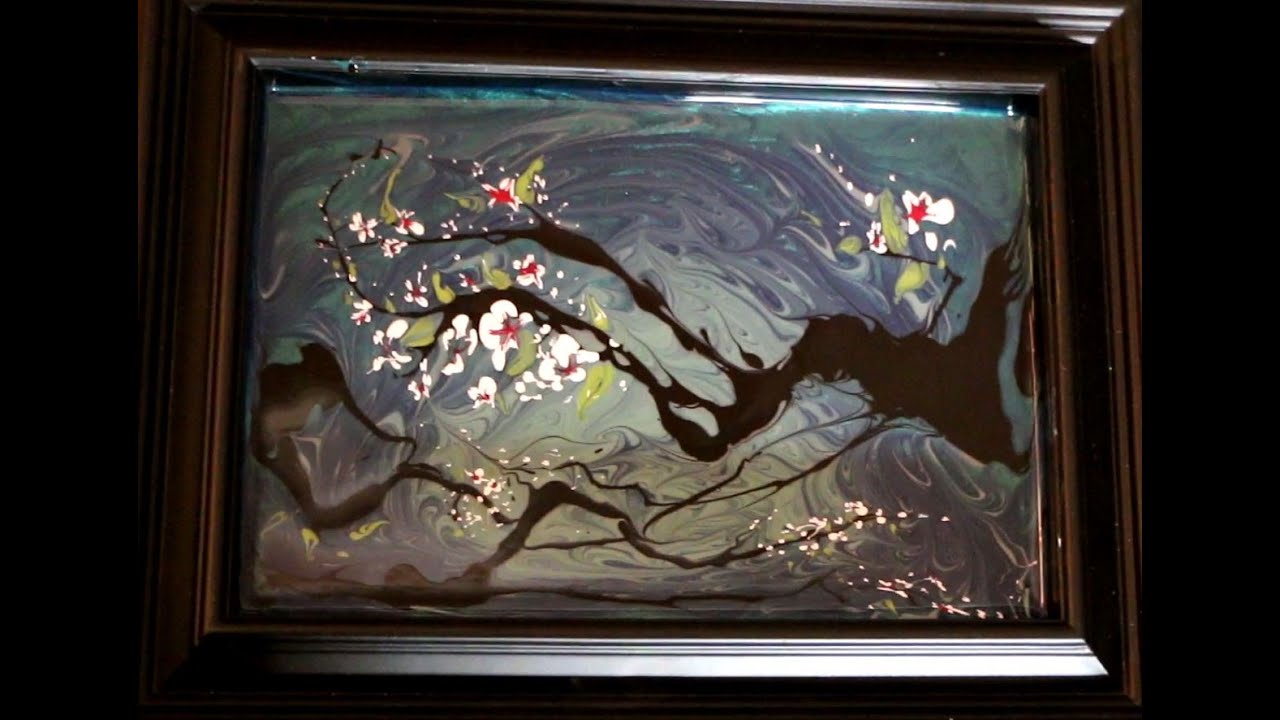The photograph showcases a beautifully framed piece of artwork set against a black background. The frame is a thick, dark brown, almost ebony or dark walnut, exuding a rich, deep tone. The artwork inside the frame seems to blend marbled ink textures on paper with a glossy finish, resembling lacquer but likely not. The background features a bluish to turquoise and medium blue-green marbled effect, adding a swirling, fluid motion to the piece. In the center, ghostly, dark brown and black ink branches twine and bleed into the backdrop. These branches are adorned with delicate white flowers, their centers a vivid red, as well as a few yellow leaves, giving the piece an ethereal, almost Asian-inspired aesthetic. The overall composition evokes a harmonious blend of natural elements and intricate detailing.